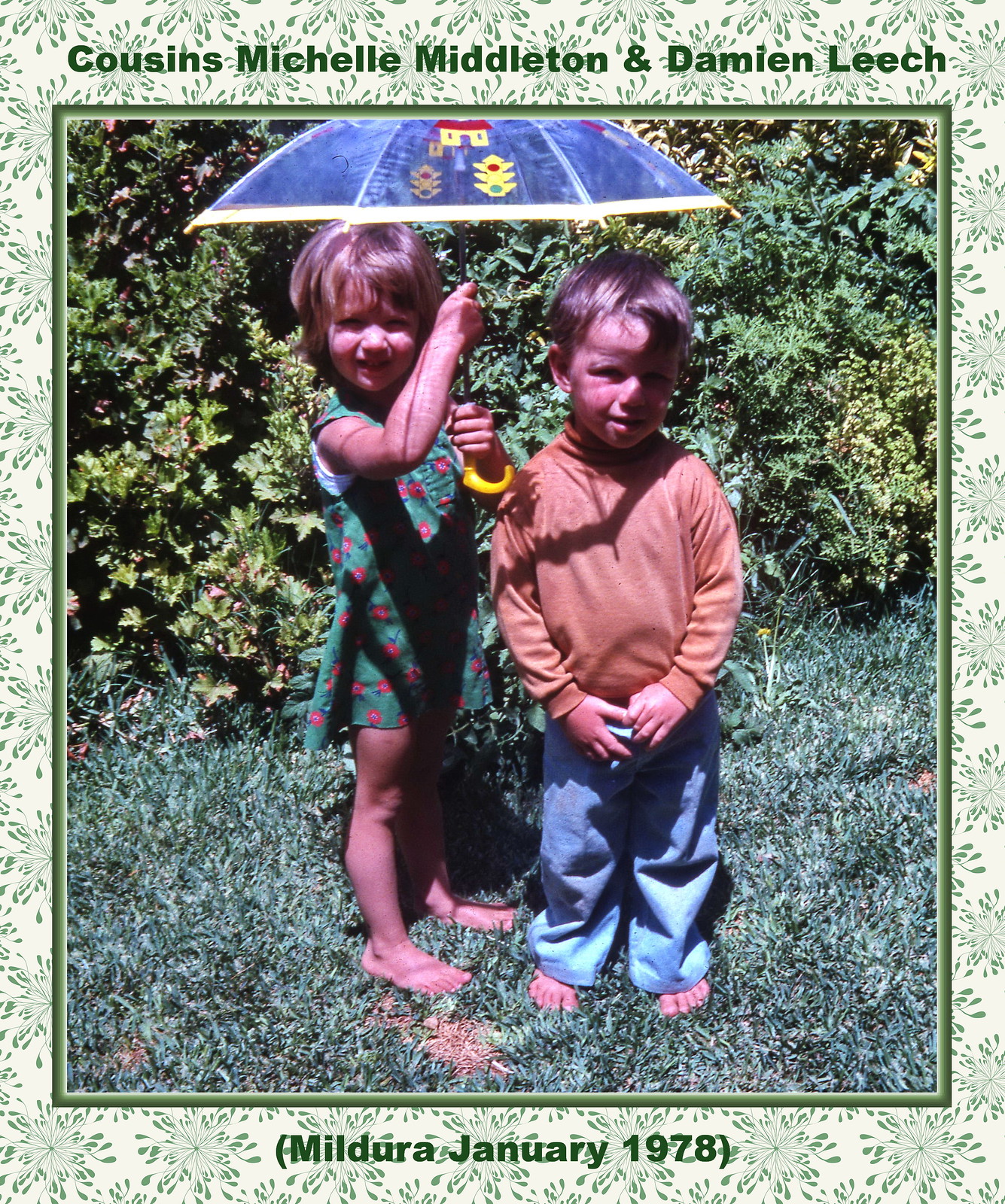This photograph from January 1978 depicts two young cousins, Michelle Middleton and Damian Leach, standing barefoot in the sun on a grassy area with shrubbery in the background. The image is framed with a green floral border. Michelle, positioned on the left, wears a green and pink sundress and holds a blue umbrella with a yellow handle over both of them. The umbrella features a drawing of a house and traffic lights. Damian, on the right, sports a peach-colored turtleneck and blue jeans. The text at the top of the photo reads "Cousins Michelle Middleton and Damian Leach," while the bottom text states "Mildura, January 1978." The entire scene captures the innocence and simplicity of childhood in the 1970s.